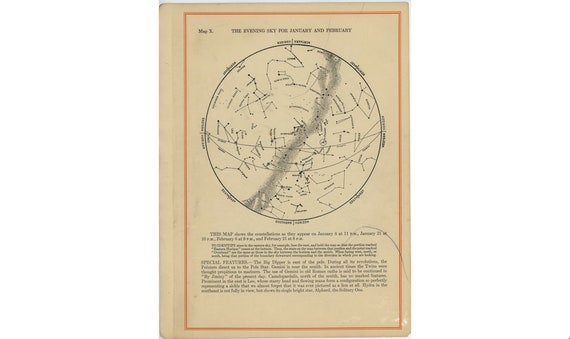This photograph depicts a page within a well-worn, aged book featuring a detailed illustration that seems to represent star constellations in a globe or circular map format. The precise details of the text are too small to decipher fully, but the visible text includes phrases like "Map X" and mentions "special features." The page is likely an interior page rather than a cover, bordered by a peach outline framing the tan background of the book. The illustration itself—rendered with pencil—depicts various constellations such as Taurus the Bull and Pisces, with connecting lines that outline these familiar celestial figures against the night sky. Text appears both above and below the circular diagram, possibly providing descriptive information about the constellations illustrated within the circle.